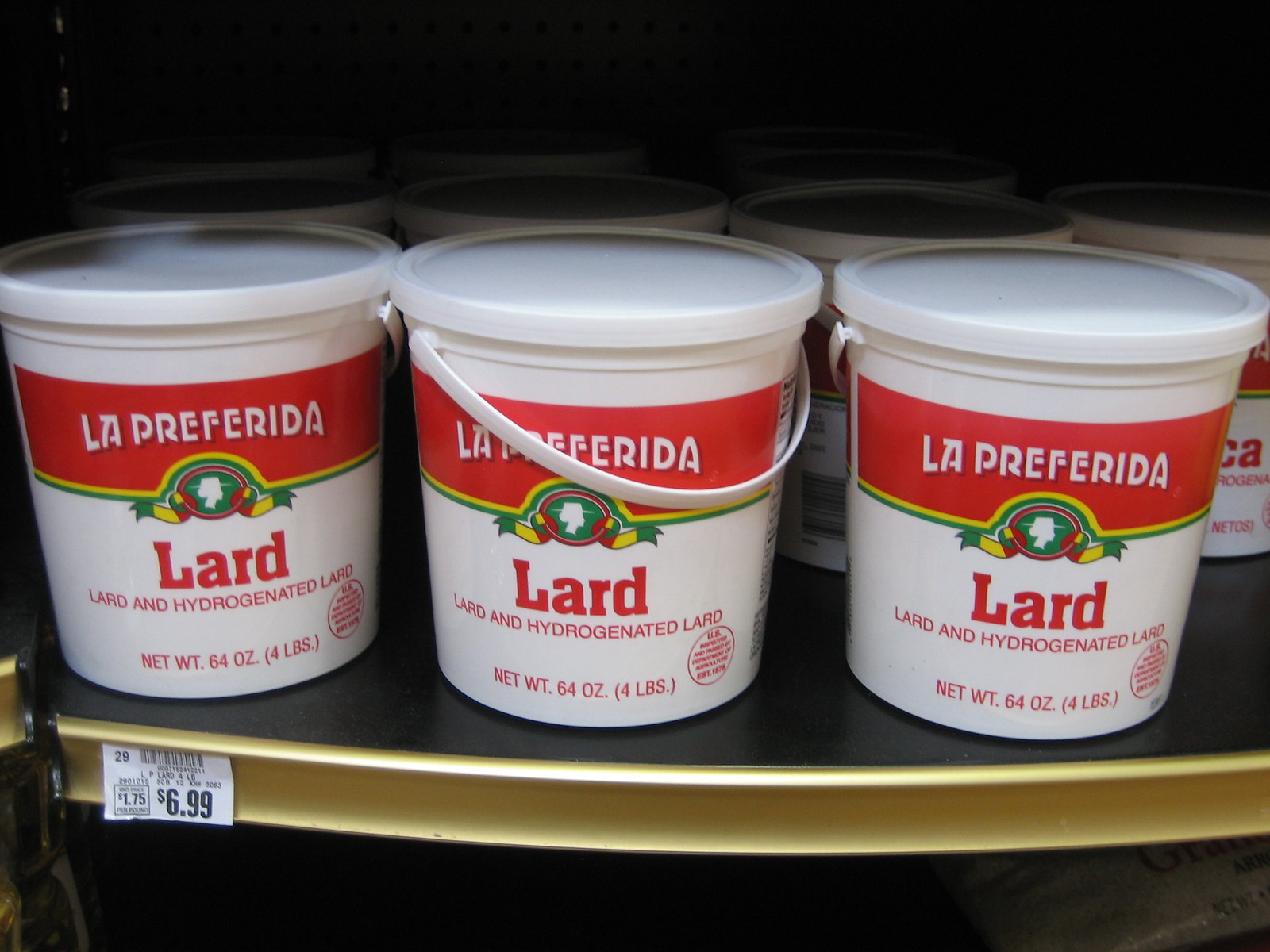The image features a large white bucket prominently placed in the center, labeled "Lard" with additional text indicating "Hydrogenated Lard" below it. This primary bucket is part of a row of identical buckets visible in the background. The entire display is adorned with a detailed, multi-colored design: a red rectangle on the left, followed by a yellow line and arch, and then a green line and arch. 

In the middle of this design is an image resembling a woman's side profile enclosed within a red circle, over a white background. Beneath this, the text "Net Weight: 64 oz (4 lbs)" is clearly visible. Also notable is a prominent red label indicating approval from the U.S. Food and Drug Administration (FDA).

The bottom shelf of the display is gold in color and features several price tags: $6.99 at the bottom left, $1.75 slightly to the left of the previous tag, $2.99 at the top left, alongside a barcode. The lower portion of the image is enveloped in dark shadows, creating a stark contrast against the brightly lit upper sections.